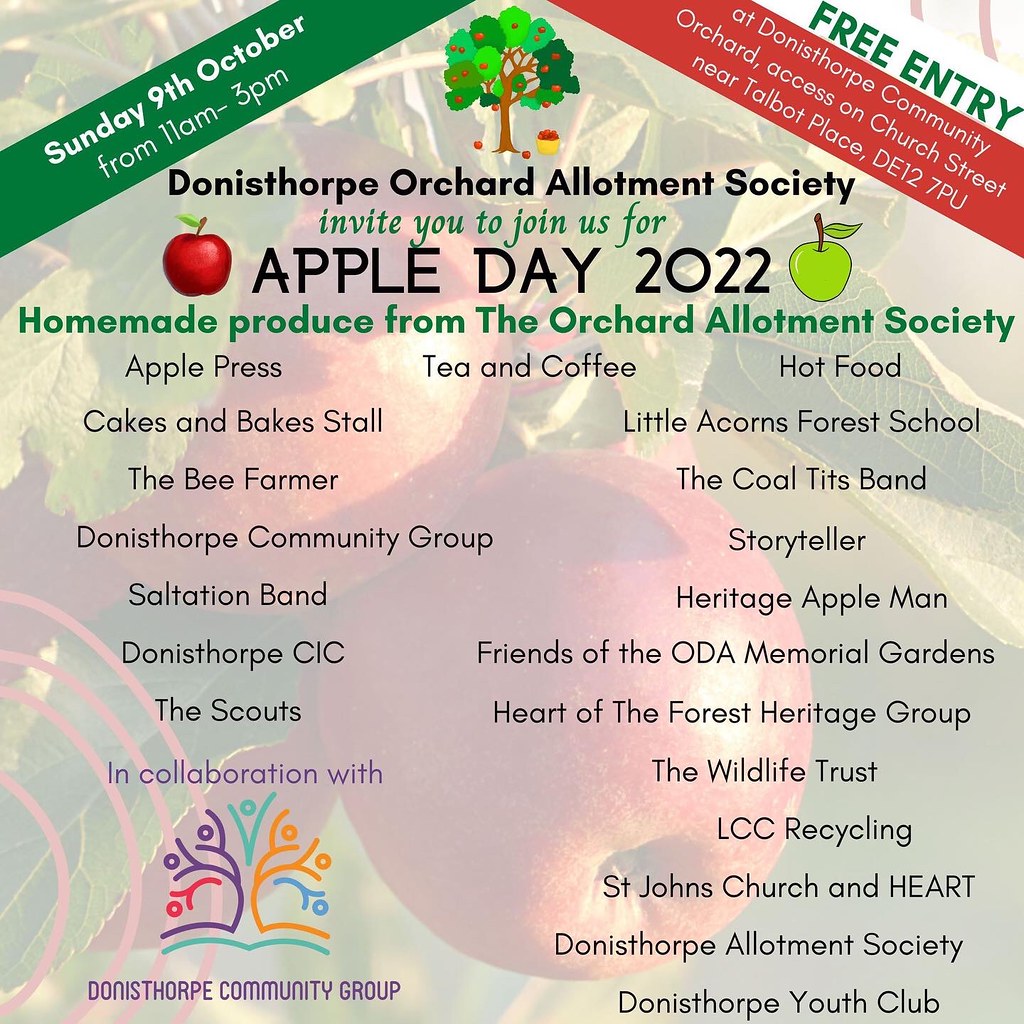This image is an advertisement for Apple Day 2022, hosted by the Donnesthorpe Orchard Allotment Society. At the top center, there's a hand-drawn graphic of a green apple tree adorned with apples, along with an apple container at its base. The background features a faded photograph of apples and leaves, creating a layered and transparent effect. 

At the top left, in green text, it announces the event details: "Sunday, 9th of October from 11am to 3pm." On the top right, it mentions "Free entry at Donnesthorpe Community Orchard, access on Church Street near Talbot Place, DE 12 7PU." 

The central part of the image bears the title: "Donnesthorpe Orchard Allotment Society invites you to join us for Apple Day 2022," followed by details of various attractions. These include homemade produce from the Orchard Allotment Society, apple press, tea and coffee, hot food, cakes and bakes stall, Little Acorns Forest School, The Bee Farmer, The Coal Tits Band, Donnesthorpe Community Group, Storyteller, Salvation Band, Heritage Apple Man, Donnesthorpe CIC, Friends of the ODA Memorial Gardens, The Scouts, Heart of the Forest Heritage Group, The Wildlife Trust, LLC Recycling, St. John's Church and Heart, Donnesthorpe Allotment Society, and Donnesthorpe Youth Club. 

At the bottom left, there is a colorful line drawing of a tree labeled "In collaboration with Donnesthorpe Community Group." The composition integrates additional images: a red apple to the left of the main title and a green apple to its right.